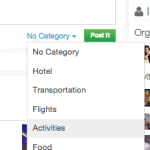The image appears to be a highly zoomed-in section of a social media site. The visible portion includes a horizontal thin gray line at the top, followed by the outline of a partial rectangle that intersects with another vertical thinner gray line, which creates a visual division on the page. Below this, there is substantial white space leading to a vertically oriented thicker gray line, adjacent to the outline of a gray avatar.

In the upper portion, the letters "O-R-G" appear in black text. There are portions of four images visible, with letters "I" placed between the first two images. It seems like part of a word is being displayed.

A white pop-up rectangle is overlaid on this section and spans downward beyond visible view. It has a gray outline and contains black text listing categories: "no category", "hotel", "transportation", "flights", "activities" (highlighted in gray), and "food", though the text extends beyond the visible area.

Behind this pop-up, in light blue text, the phrase "no category" is partially visible with a downward-pointing light blue triangle next to it. Below this is a green rectangular box with white text reading "Posted" with a capital "P" and "I". Additionally, three horizontal gray lines are visible in the background but are partially obscured by the pop-up.

In summary, the image captures part of a social media platform's interface, specifically highlighting a segment where a user is likely interacting with items listed under various categories, with "activities" being the currently selected category. The presence of overlapping elements and cutoff text suggests a layered, zoomed-in view that focuses more on the site's structural layout than on its complete content.